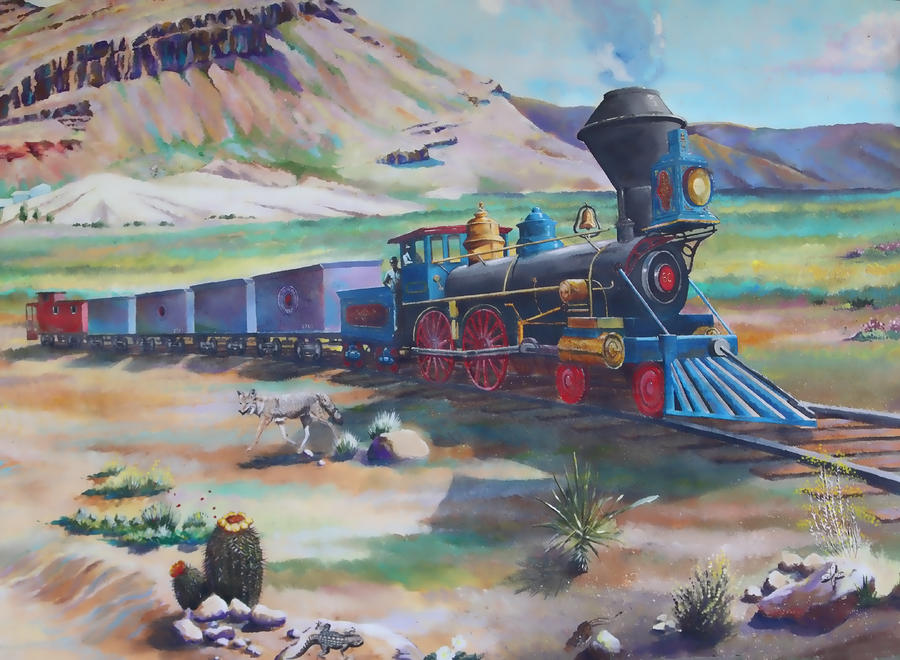This painting depicts a vibrant steam engine train traversing a railway line set in a semi-arid landscape adorned with greenery, including bushes, plants, and cacti. The train, with its black engine featuring a blue cattle guard at the front and red wheels, prominently emits steam from a smokestack. Following the engine are several cars, with the middle compartments painted blue and the last car being a red caboose. The train glides over wooden tracks, while a gray coyote or wolf walks in the foreground. The backdrop includes a mountain range with geological formations reminiscent of the Grand Canyon, showing signs of erosion. A bright blue sky stretches above, enhancing the scene’s vivid colors. Small green plants and patches of brown soil detail the ground alongside the railway line.